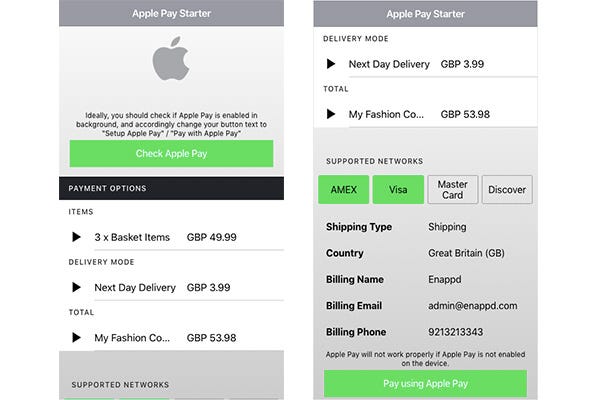This image presents a comparison of two distinct sections of a website, side-by-side, each separated by a white border.

### Left Side:
- **Top Border:** 
  - *Background Color:* Dark gray
  - *Text:* "Apple Pay Starter" in white.
- **Main Section:** 
  - *Background Color:* Light gray
  - **Middle:**
    - *Centered:* Apple icon 
  - **Below the Icon:**
    - Three lines of informational text.
    - *Green Tab:* Spans the width, labeled "Check Apple Pay" in white text.
- **Lower Sections:**
  - *Black Border:* 
    - *Text:* "Payment Options" in white.
  - **Options List:**
    - *First Option:* Details the number of items in the basket and their total price.
    - *Second Option:* Describes the delivery type and its associated cost.
    - *Total:* Displays the overall total.
  - **Bottom Section:**
    - *Color:* Gray
    - *Bottom Left Corner Text:* "Supported Networks" in black.

### Right Side:
- **Top Border:** 
  - *Background Color:* Dark gray
  - *Text:* "Apple Pay Starter" in white.
- **Main Section:**
  - **First Box:**
    - *Background Color:* White
    - *Text:* "Delivery Mode" in black.
  - **Second Box:**
    - *Background Color:* White
    - *Text:* Displays the total.
  - *Below Text Area:* 
    - *Background Color:* Gray
    - *Text:* "Supported Networks" in black.
- **Supported Networks:**
  - *First Two Tabs:*
    - *Color:* Green
    - *Text:* "Amex" and "Visa" in black.
  - *Next Two Tabs:* 
    - *Color:* Gray
    - *Text:* "MasterCard" and "Discovery" in black.
- **Form Fields:**
  - List on the left showing:
    - Shipping type, country, billing name, email, and phone.
  - *To the right:* Corresponding input fields.
- **Bottom Section:**
  - *Color:* Green
  - *Text:* "Pay using Apple Pay" in white, spanning the entire width of the section.

This detailed comparison highlights the various elements and design details of each section, allowing for a clear understanding of their layout and functionality.